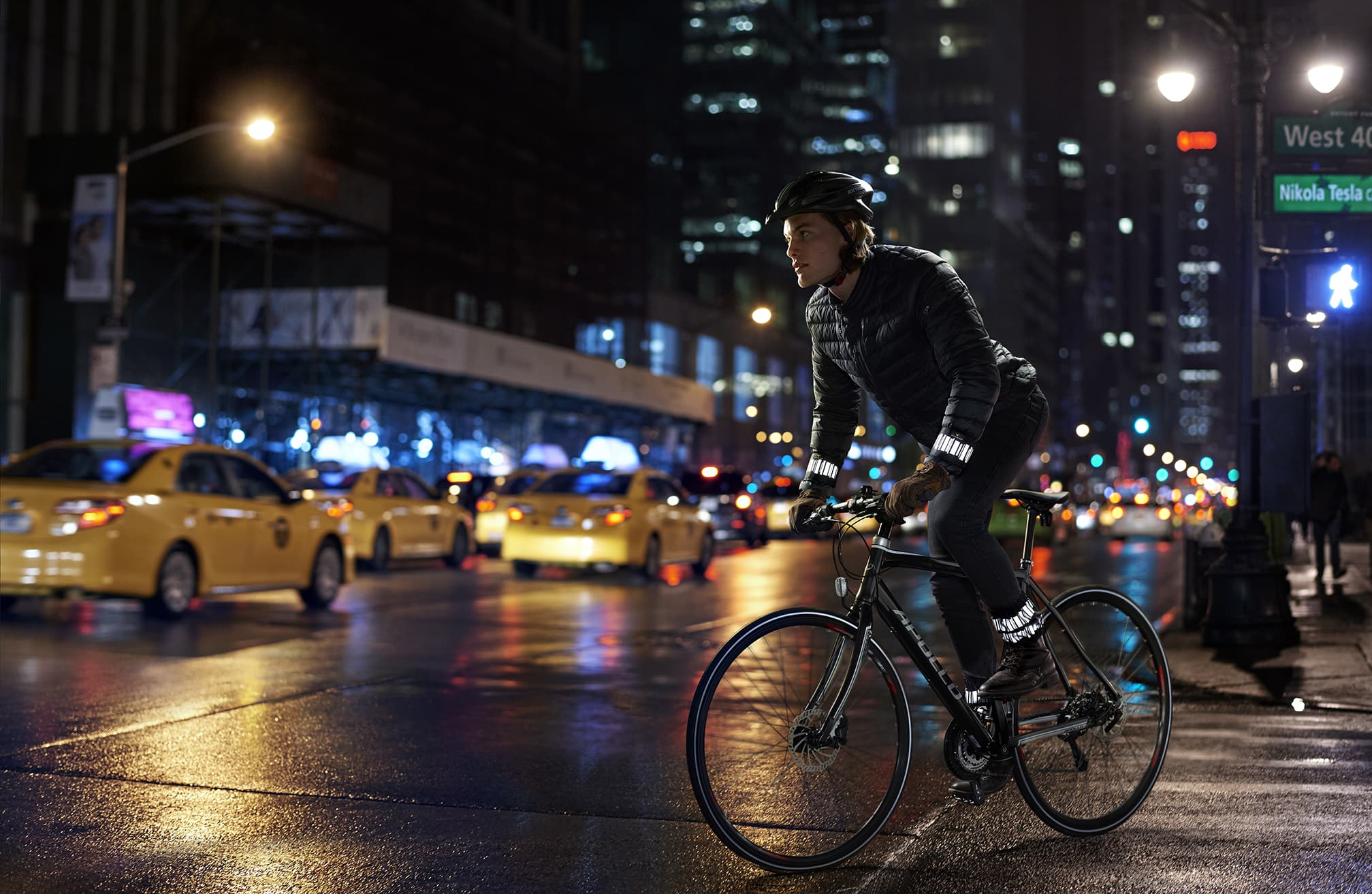In this nighttime photograph set in a bustling cityscape, a young man of European descent rides a sleek, black bicycle at the forefront in the right-hand corner of the image. He is clad in a black helmet, black jacket, and black pants, with shining reflectors affixed to his wrists and ankles. The wet, slick streets hint at recent rain, reflecting the myriad lights from street lamps, traffic signals, and the surrounding buildings. A street sign to the right reads "Nikola Tesla" and "West 40," placing the scene in Manhattan. To the left, a long queue of yellow taxis waits in traffic, their taillights glowing red further down the road, which fades into a blur of lights and towering skyscrapers in the background.